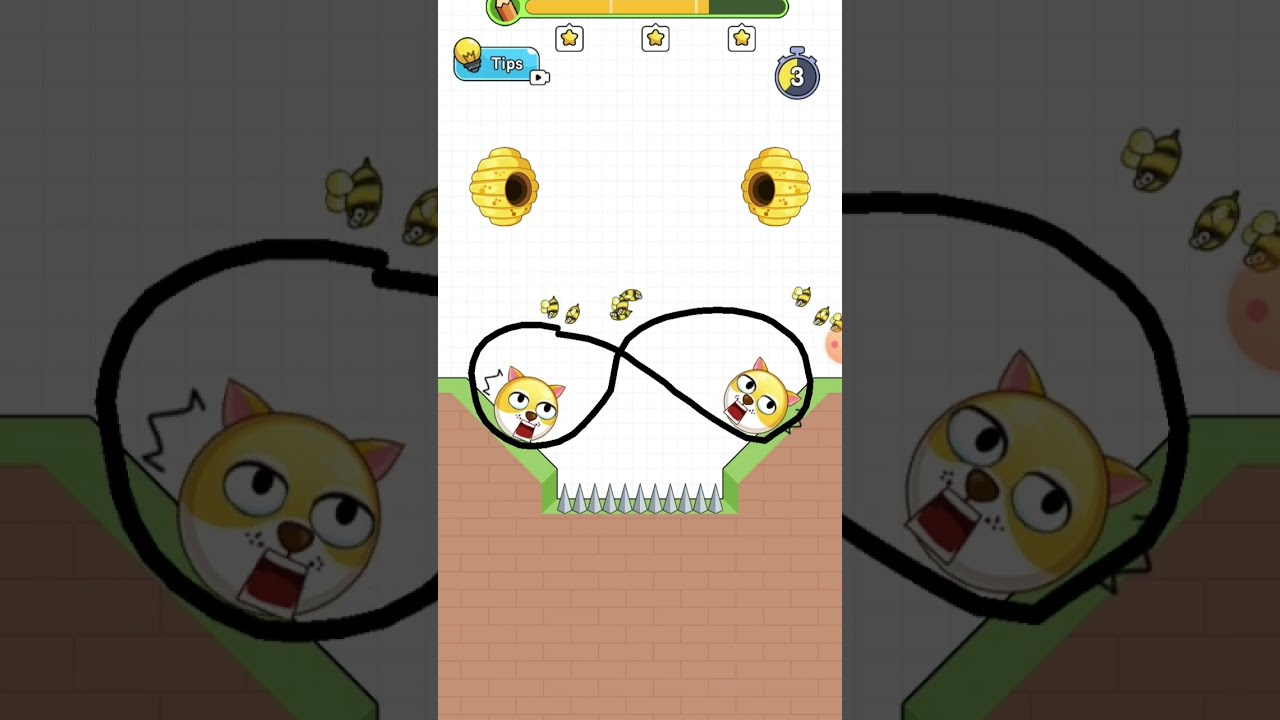In the middle of a smartphone screenshot, there is a large, rectangular image dominated by two circular cat heads. The heads are yellow on the top half and white on the bottom half, featuring gaping, rectangular mouths, brown noses, and little pink ears. The backdrop is slightly darkened, emphasizing the vibrant color scheme of the characters. Surrounding the cats is a grassy landscape that tapers downward to reveal a bed of spikes directly below them. Hovering above the cats are bees, with beehives positioned above each head. The scene is framed by several in-game UI elements: on the top left corner, a light bulb icon labeled "Tips," a star bar with three stars around a house icon at the top center, and a stopwatch showing the number three at the top right. The image appears cartoonish, vibrant with colors like yellow, blue, orange, green, brown, and gray, suggesting it's a screenshot from a mobile video game.